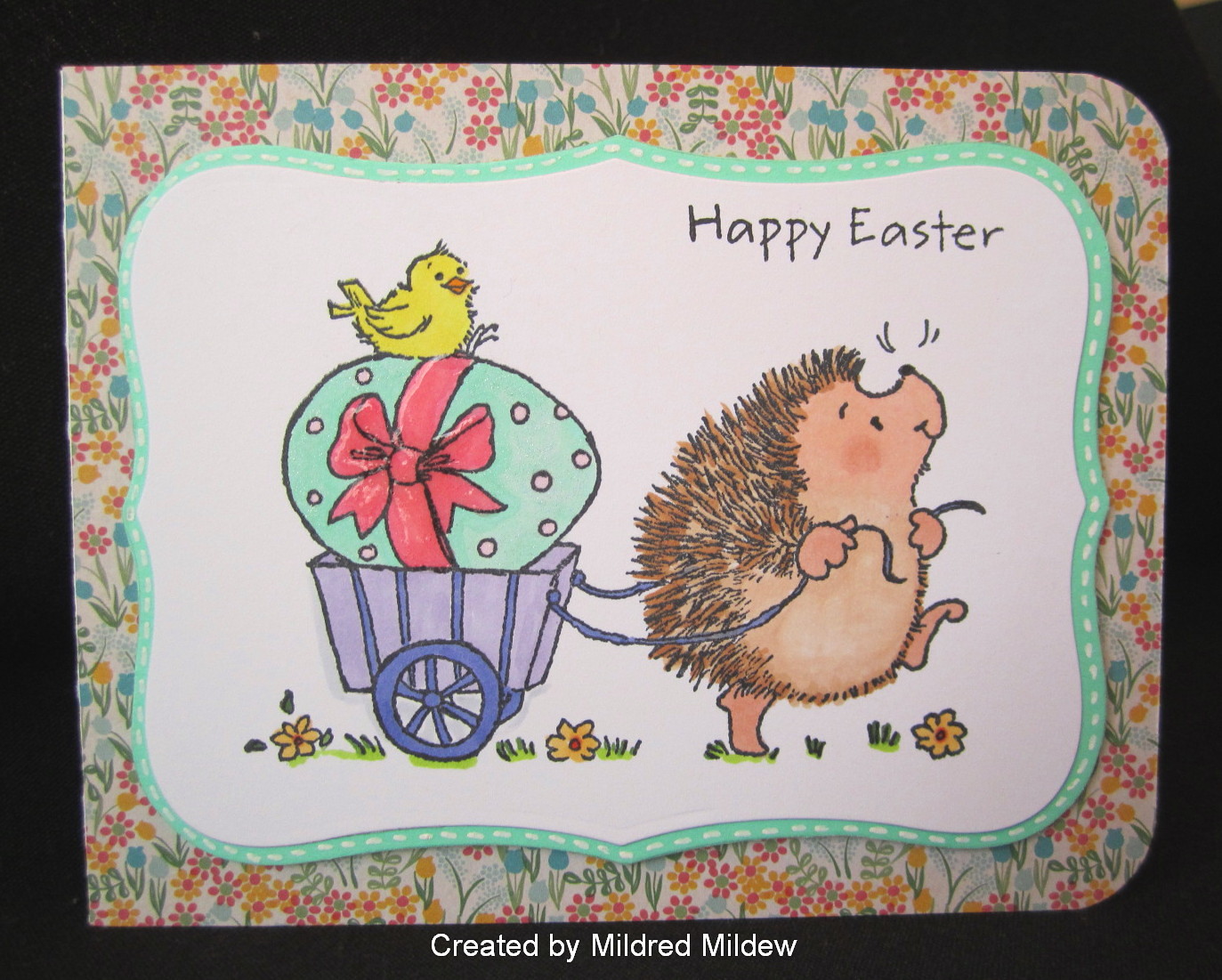The image depicts a charming Happy Easter card with a whimsical scene. At the center of the white background is a joyful brown porcupine standing upright and pulling a two-wheeled, striped purple wagon with a great big smile on its face. Inside the wagon rests a large, pastel green egg adorned with a pink ribbon, atop which perches a cheerful yellow chick with an orange beak. The ground is decorated with sprigs of grass and colorful flowers. The card is bordered with wavy lines and features a beige background adorned with red, yellow, and blue flowers with green stems. The upper right corner of the card reads "Happy Easter" in black letters, and at the bottom, the text "Created by Mildred Mildew" is written in white. The card has a rounded edge on one side and a black rectangular frame surrounding the image, creating a delightful and festive visual.